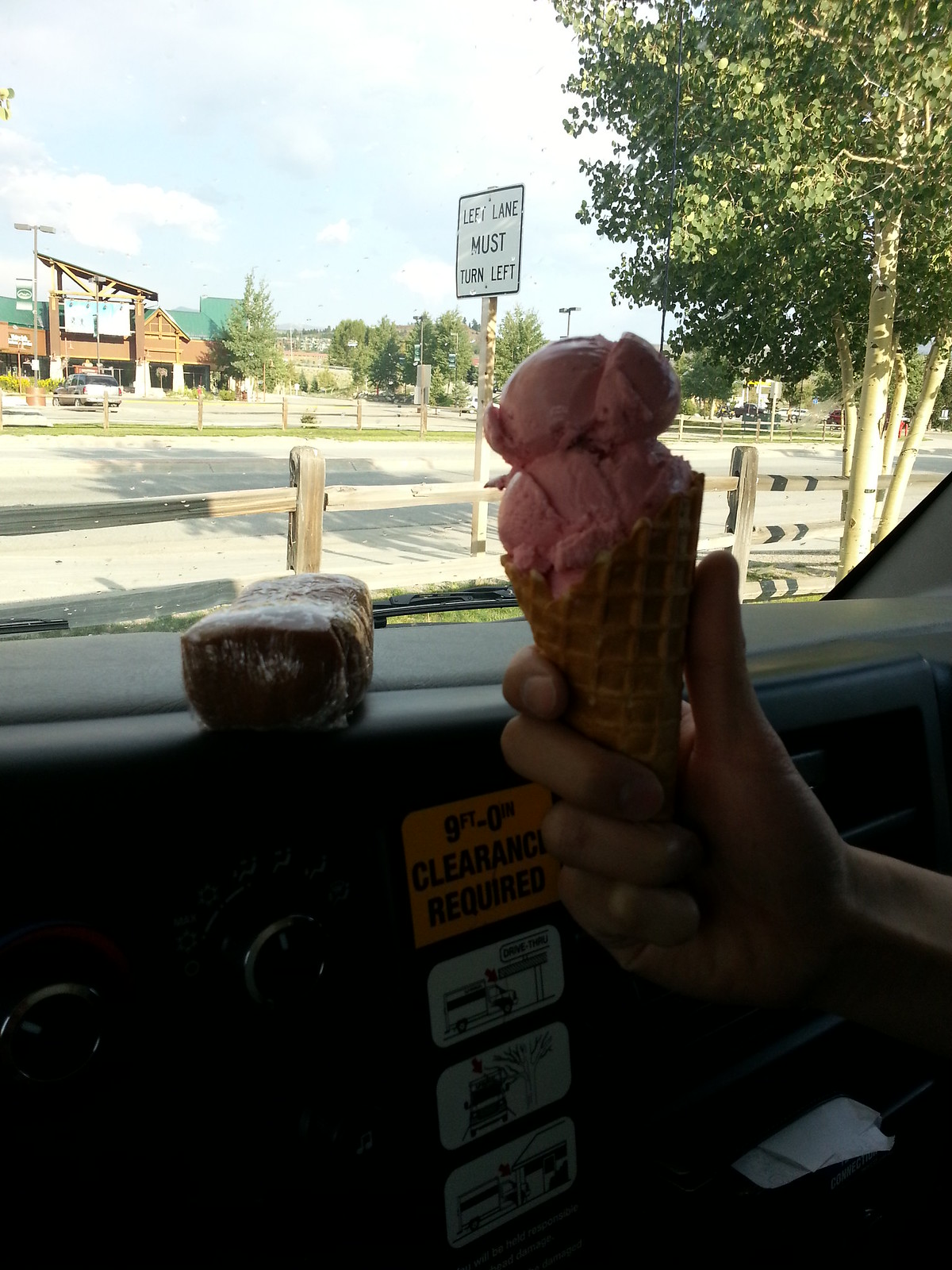In this image, we see the interior of a U-Haul truck, identifiable by the orange sticker on the dashboard that reads "Nine feet, zero inches clearance required" along with three illustrative stickers depicting the truck getting stuck under low-clearance obstacles. A right hand is extended into the center of the frame from the right, holding a waffle cone with two scoops of pink ice cream, possibly strawberry or cherry flavored. To the left on the dashboard lies a piece of fudge wrapped in plastic. Through the window, we observe a largely empty parking lot bordered by a rustic wooden fence and a tree in the right corner. Across the street, there's a building with a green roof and wooden façade, likely part of a shopping center. A sign in front of the truck reads "Left lane must turn left." The sky is somewhat cloudy, indicating it is daytime.